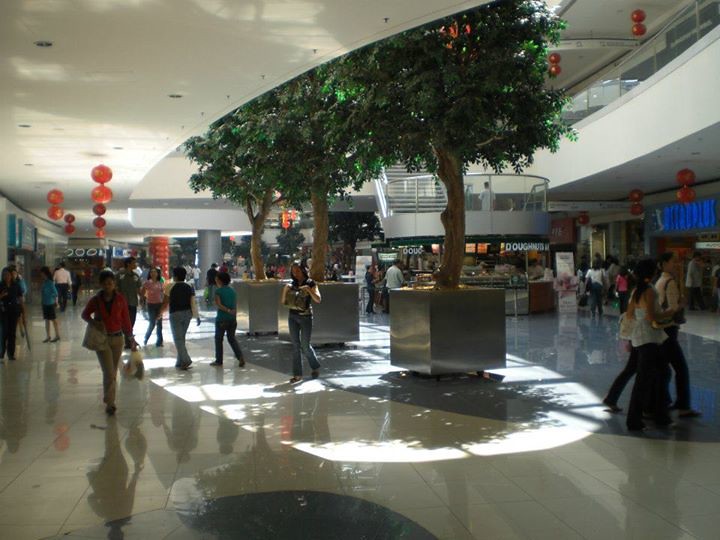This image captures the bustling atmosphere inside a multi-level indoor shopping mall, possibly located in Asia. The bustling scene on the bottom floor shows dozens of people, some carrying shopping bags, indicating a busy shopping day. Visible on both the left and right sides of the image are various shops, with a central donut kiosk prominently featured. The floor's shiny white and blue vinyl tiles reflect the ambient light.

A stairway in the background leads to the second level of the mall, which features a balcony area allowing visitors to look down at the activity below. The second floor is also home to a sunroof, from which sunlight filters through, highlighting three massive potted trees. These trees, which might be artificial, stretch from the ground floor upwards, their leaves casting intricate shadows on the tiled floor.

Adding to the vibrant ambiance, numerous red lanterns hang from the ceiling, suggesting cultural decor, possibly linked to Asian festivities. Despite the somewhat low lighting, the sunroof's natural light creates a lively and inviting atmosphere. The people, a mix of possibly White and Asian individuals, navigate through the mall, which may also house a food court, indicated by the presence of the donut store signage. This detailed scene paints a vivid picture of a dynamic and lively shopping mall experience.